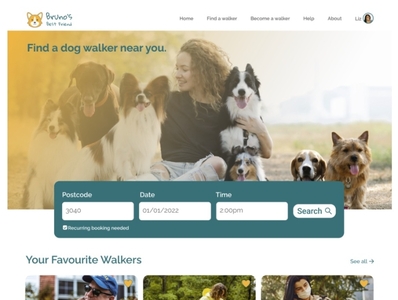The image showcases a webpage from a service named "Bruno's [incomplete text]." At the top of the page, there are several blurred menu options labeled as "Home," "Help," and "About," with additional unreadable options. Below the menu, there is a prominent section featuring a photograph of a woman sitting on the ground, surrounded by seven different dogs who are playing with her. Captioned with "Find a dog walker near you," this section aims to engage pet owners seeking local dog walking services.

Beneath the image, there's a grayish-blue input box with fields for a postcode "3040," a date set to "01/01/2022," and a time "2 p.m." Accompanying this input area is a search button to help users find available dog walkers within their specified criteria.

Further down, there is another section titled "Your Favorite Walkers," displaying three cropped images. The first image on the left features a man wearing glasses and a blue baseball cap. The middle image only shows a scene of trees and bushes. The details of the third image are unspecified.